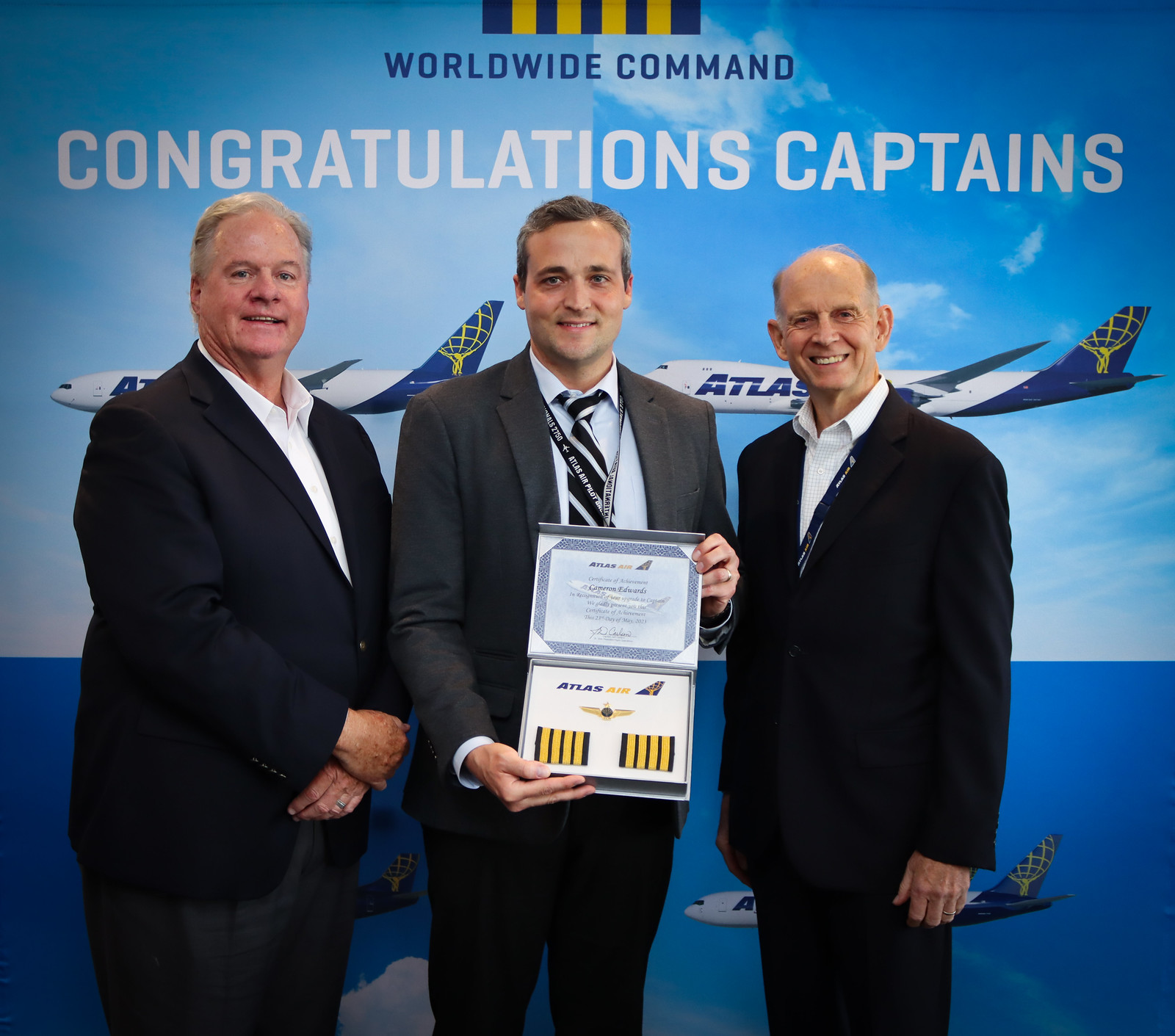In the photograph, three men stand proudly in front of a large billboard adorned with congratulatory messages and images. The backdrop features a sky-blue and yellow design at the top and reads "Worldwide Command" in bold blue letters, followed by "Congratulations Captains" in crisp white letters. Below, the poster displays several Atlas Airlines planes, recognizable by the blue and white color scheme and the iconic gold Atlas symbol on the tail fin. The background transitions into a dark blue towards the bottom, framing the men from behind.

From left to right, the first man sports a blue suit coat, white shirt, and gray pants. He has short gray hair and stands with his hands clasped in front, offering a slight smile. The man in the center holds a two-part certificate, likely an award for his achievement as a captain. Dressed in a gray suit with a light shirt and striped tie, he has short dark hair and a broad smile. Around his neck hangs another award, partially obscured by the certificate he proudly displays. The third man, on the right, wears a dark suit with a white shirt and dark pants. Slightly turned to the left, he has minimal gray hair, is balding, and beams at the camera.

The setting, possibly indoors as part of a photo shoot campaign, captures the celebratory moment of these captains recognized for their accomplishments at Atlas Airlines.